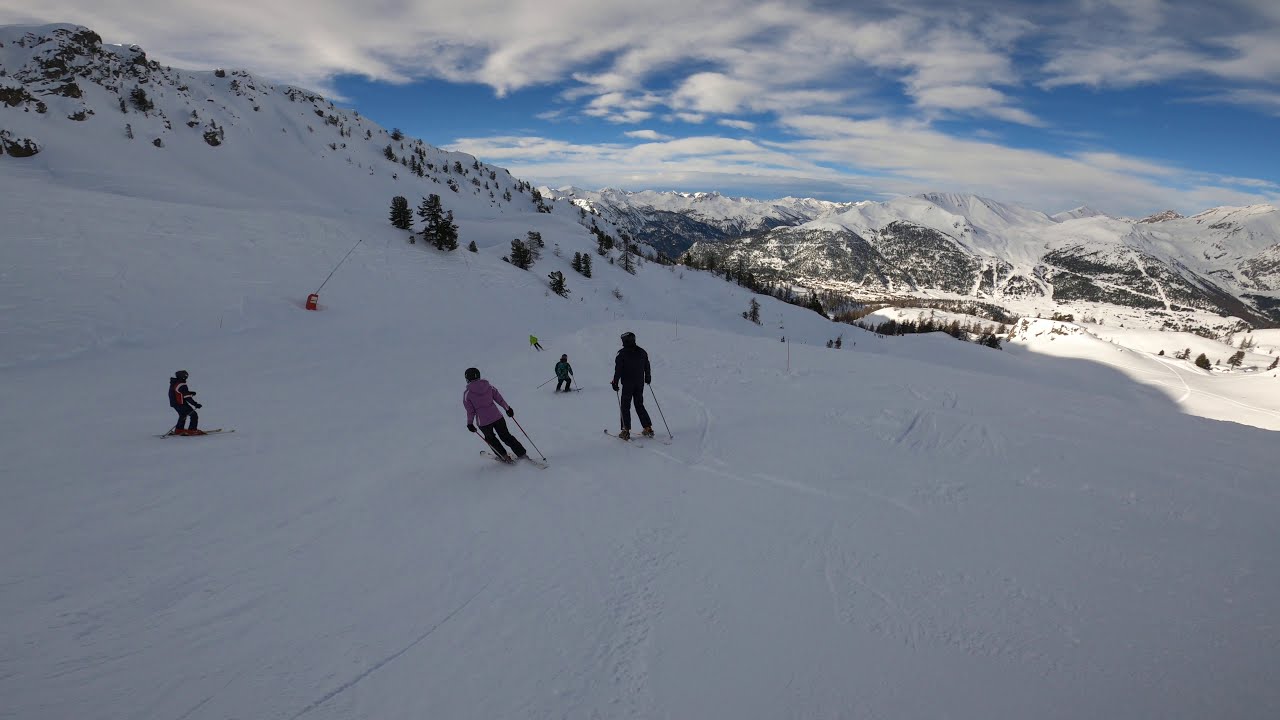This high-quality, outdoor photograph, taken during the daytime, captures a bustling ski resort with a vast expanse of white snow on a mountain slope. The ground is sloping downward with numerous people skiing across the terrain, all dressed warmly for the cold weather. The closest skier is a woman in a pink jacket and helmet, skiing with long pants on. To her right, a man in all black is also on skis, and just below them appears to be an instructor, wearing a jacket and possibly snowboarding without poles. A few more skiers are scattered across the slope, some very small in the distance. The snowy ground is shaded in large portions, yet the right side brightly reflects the sun's shine, indicating the presence of sunlight. Dotting the landscape are green trees emerging from the snow. The upper left of the photograph reveals a vast expanse of mountains, snowy at the top and darker further down, beneath a bright blue sky adorned with fluffy white clouds. The overall image is brightly lit with natural light, offering a clear and vivid depiction of a bustling ski resort.